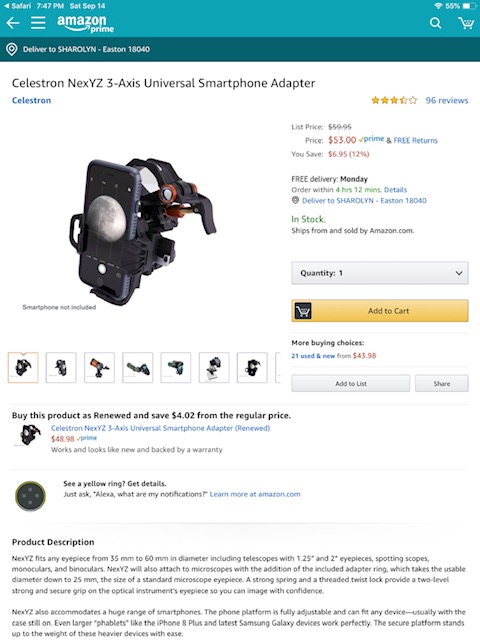Screenshot of an Amazon Prime shopping page taken at 7:47 p.m. on Saturday, September 14th. The top left corner shows the "Safari" browser, while the top right corner displays the Wi-Fi signal strength, a 55% battery indicator, a magnifying glass icon, and a shopping cart icon that contains no items.

The item being viewed is the "CELESTRON NexYZ 3-Axis Universal Smartphone Adapter," which has a rating of 4.5 stars from 96 reviews. The listed price is $59.95, currently discounted to $53 with Amazon Prime, offering free returns. This means a savings of $6.95, approximately 12%. If ordered within the next 4 hours and 12 minutes, free delivery is available by Monday. Delivery is addressed to Sharon Sherilyn Easton, postal code 81804.

The product is in stock and ships from and is sold by Amazon.com. The default quantity is one. Below the main product details, several images of the adapter are displayed. There is also an option to purchase a renewed version of the product for $48.98, saving an additional $4.02, which is also available with Amazon Prime. A yellow ring provides further details, and users are prompted to ask Alexa for their notifications.